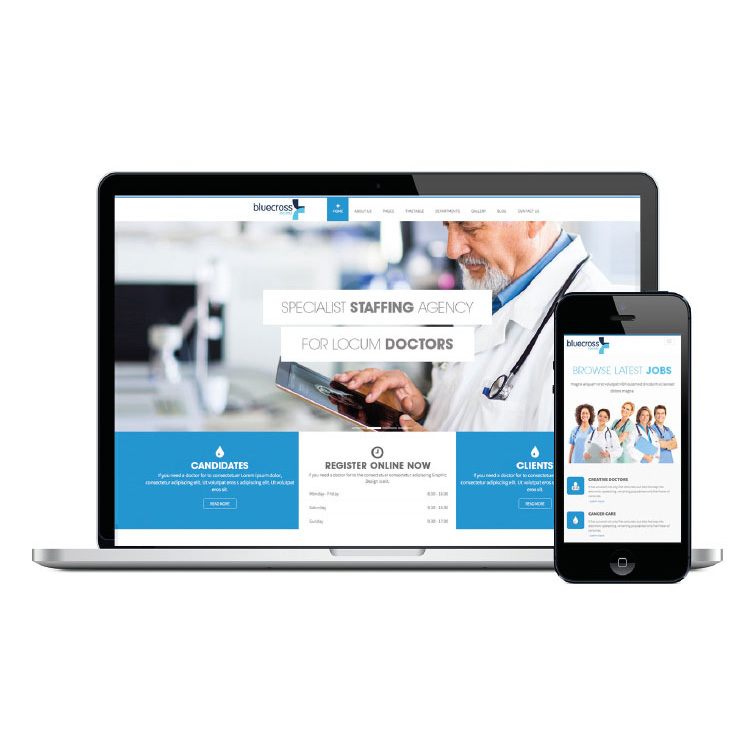The image features a website displayed in two formats: on a generic laptop and on a smartphone. The website is associated with Blue Cross and prominently showcases its home page. The larger image on the left displays the home page on a laptop. Toward the top two-thirds of this display is an image of a white man dressed like a doctor, wearing a lab coat with a stethoscope around his neck, and looking down at a tablet. The caption above reads, "Specialist Staffing Agency for Locum Doctors."

At the bottom of the laptop screen, there is a horizontal section of text. The first box on the left, highlighted in blue, features the word "Candidates," but the smaller text below it is unreadable. Adjacent to this, there is an icon of a clock followed by text on a white background that says, "Register Online Now," with additional unreadable text underneath. To the right, there is another blue box labeled "Clients," with similarly unreadable text beneath it.

On the right side of the image, a smartphone also displays the Blue Cross home page. It features the phrase, "Blue Cross, Browse Latest Jobs." The top of the phone screen shows an image of four white medical professionals—three women and one man—dressed in either lab coats or scrubs, all with stethoscopes. Below this, there are two more blocks of text, which are again too small and blurry to decipher.